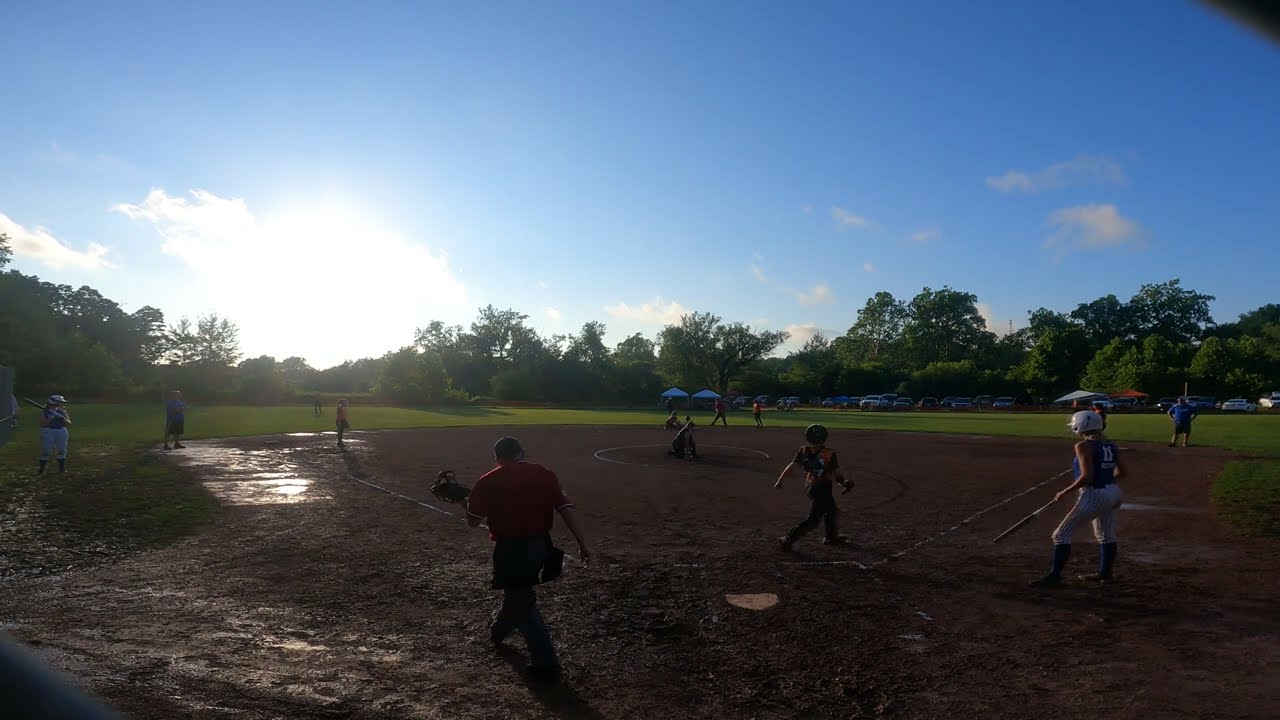An outdoor little league softball game is underway on a muddy, wet baseball field that glistens under a partly sunny sky. The field’s brown dirt is marked with white lines demarcating the various areas of play and bases. Puddles of water can be seen on the left side of the field, a testament to the recent rainstorm. Standing prominently in the center of the image is a figure in a red polo with white trim, gray pants, and a black apron, holding a black protective face mask, clearly the umpire. Players are scattered across the field, including a young girl preparing to bat. The background features parked cars in a lot, several umbrellas, and a dense, forest-like area of tall trees under a light blue sky with white clouds. The setting is daytime, marked by the subtle sunshine breaking through the clouds, and suggesting little spectator presence due to the weather.